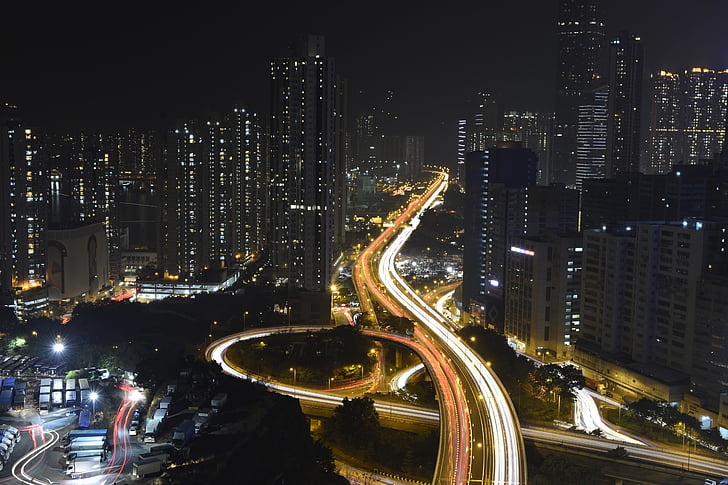An aerial view of a bustling city skyline at night reveals a vibrant, fast-paced urban landscape. Cutting through the heart of towering skyscrapers, a four-lane freeway glows brightly, its neon-like trails of red and white headlights streaking in both directions, indicating continuous, high-speed traffic. The skyscrapers on both sides of the freeway are illuminated, each floor and room contributing to the mosaic of yellow and white lights that define the city's nightscape. Some buildings, further off in the distance to the right, remain dark. In the bottom left corner, a parking lot filled with parked tractor-trailers and pickup diesel trucks adds to the urban complexity, while more unique structures and additional streets of light weave through the bottom right. The photograph, capturing the essence of a lively, illuminated city, has a distinctly surreal quality, possibly enhanced by the photographer to emphasize the city's dynamic energy.